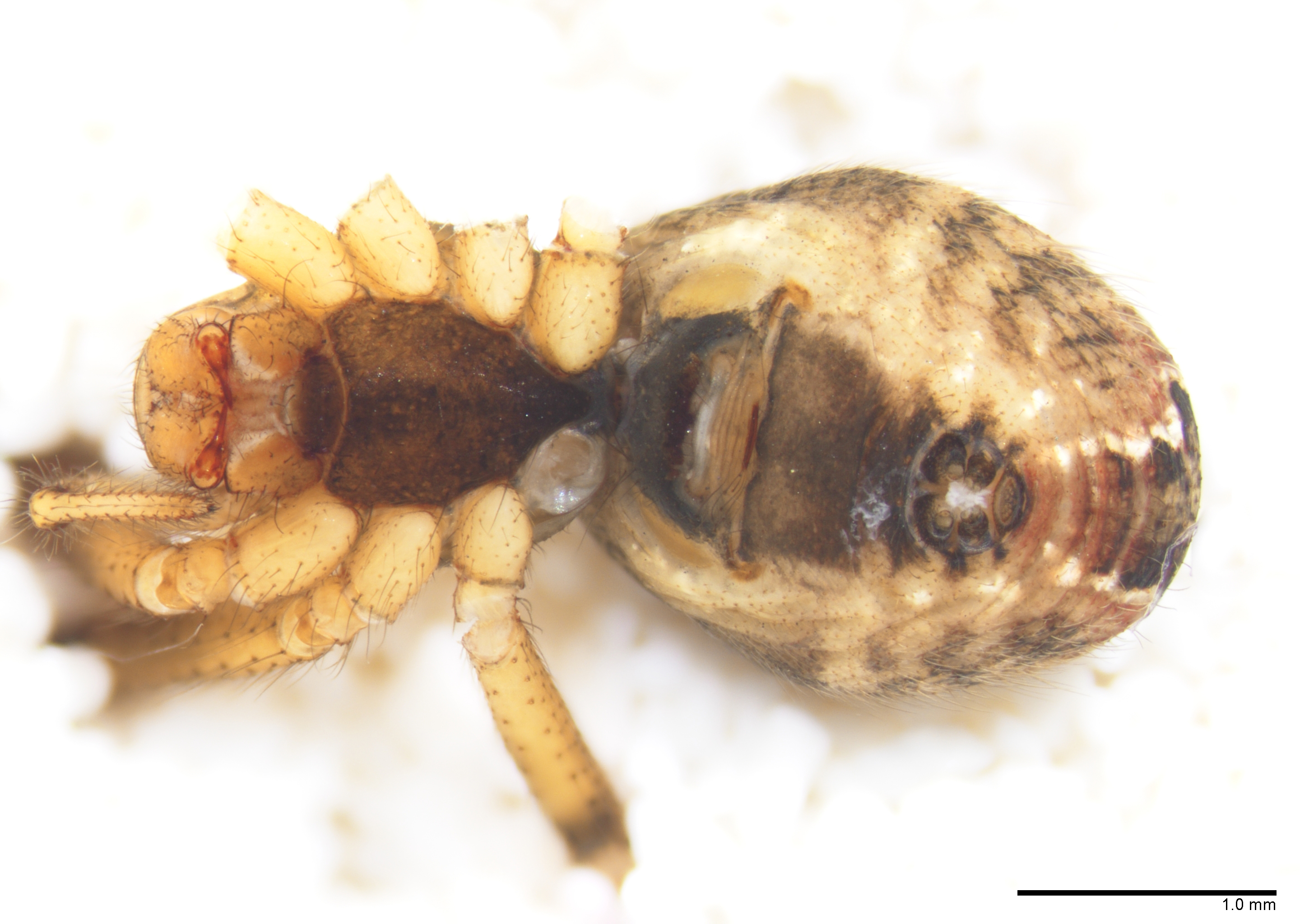This is a detailed close-up photograph of a spider, predominantly brown in color with varying shades. The spider's body features a dark brown central area, with lighter brown extending towards the sides and legs, all of which exhibit fine hairs. Notably, the spider appears to be injured, with several legs missing; only three remain intact on the spider's left side, while the right side shows remnants where legs have been lost. The spider has striking red or orange-colored eyes that stand out against the brown hues of its body. The background of the image is stark white, peppered with small brown dots surrounding the spider. At the bottom right corner of the photograph, there is a small horizontal black line annotated with '1.0 mm,' providing a scale for the image. The spider is oriented head towards the left, and tail pointed to the right, giving a slightly upside-down perspective. There seems to be an element, potentially a screw, intersecting the top part of the spider in the image, suggesting it might be a mounted or digital illustration.